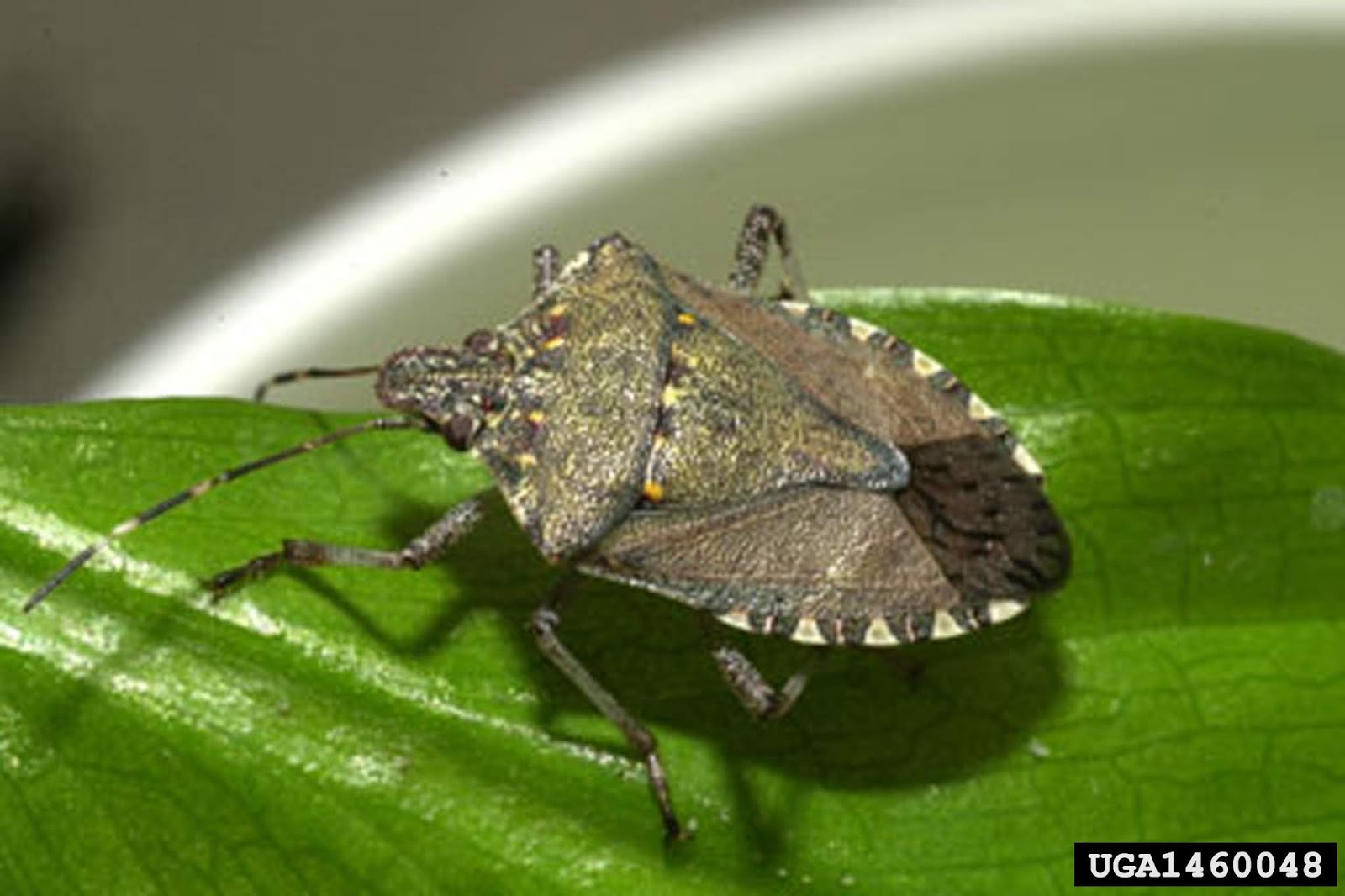This highly detailed macro photograph captures a beetle, possibly a stink bug, in a striking close-up against a blurred background. The rectangular image features a vibrant green leaf, which spans horizontally across the lower half of the frame. The leaf is meticulously detailed, showcasing distinct light green vein lines. The background shifts from dark gray on the left to a lighter gray toward the center, creating a subdued, out-of-focus backdrop that accentuates the sharply defined subject.

Centrally positioned on the leaf, the beetle's oval body extends into a tapered rear end. Its hard shell displays a mosaic of dark browns and grays, adorned with a series of small white triangles along the edges. The insect has three legs on each side of its body, and just past its front two legs, there is a notable triangular marking that points toward its tail. The beetle's head, which is brown with yellow spots, is equipped with two long, black and white antennae, and slender, brown arms.

Noteworthy details on the beetle's shell include a brown-colored fin-like structure near the rear and a central area that is a lighter, greenish-brown hue with yellow trimming. Additionally, the bottom right corner of the image contains a black strip with white text that reads "UGA 1460048," possibly indicating a reference or catalog number from the University of Georgia.